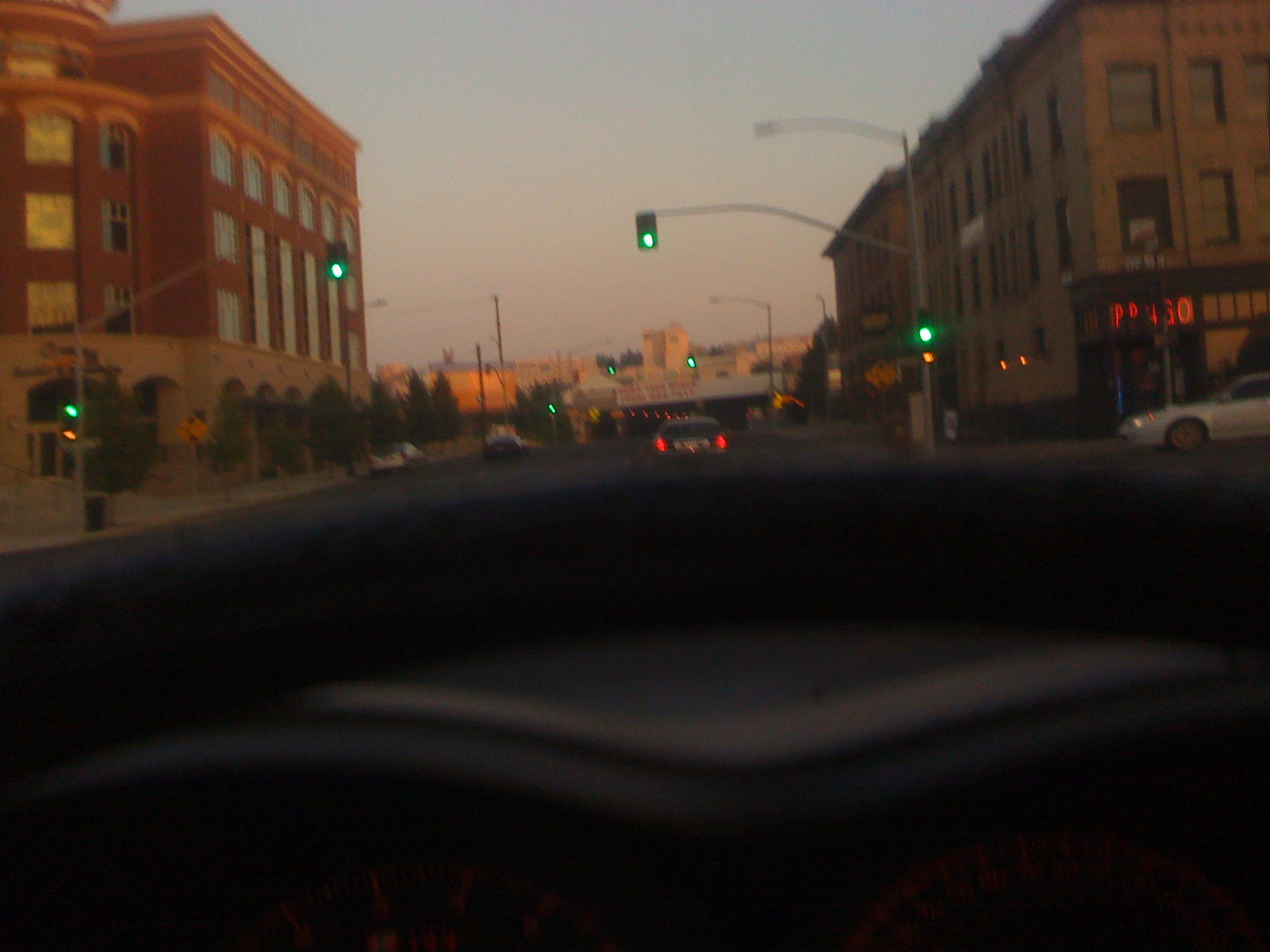This photograph appears to be taken from the driver's seat of a vehicle, capturing a road scene framed by a dashboard. The dashboard is black, and you can discern gauges at the bottom left and right. The view through the windshield shows the main road ahead, which is dark gray or black, lined with several moving and stopped cars. A white car is seen pulling out to the right, while another car ahead has its brake lights on. Above, traffic lights fixed to dark gray poles display green lights, echoed by similar lights visible in the distance.

Flanking the road, two large, red brick buildings with numerous windows and a gray arch flanked by mid-height evergreen trees sit on the left. Both buildings appear to be apartment complexes, about three stories tall. To the right, another red building and a partially visible neon sign, featuring red lettering with the discernible characters "P" and "G-O," adds to the city's ambiance. The photograph captures a sky with patches of blue and spots of white, giving the impression of a day with scattered clouds. Adding a touch of early morning or evening mood, the scene is bathed in a soft golden hue. In the distance, a tunnel-like structure illuminated by lights can be seen, hinting at the continuation of this urban journey.